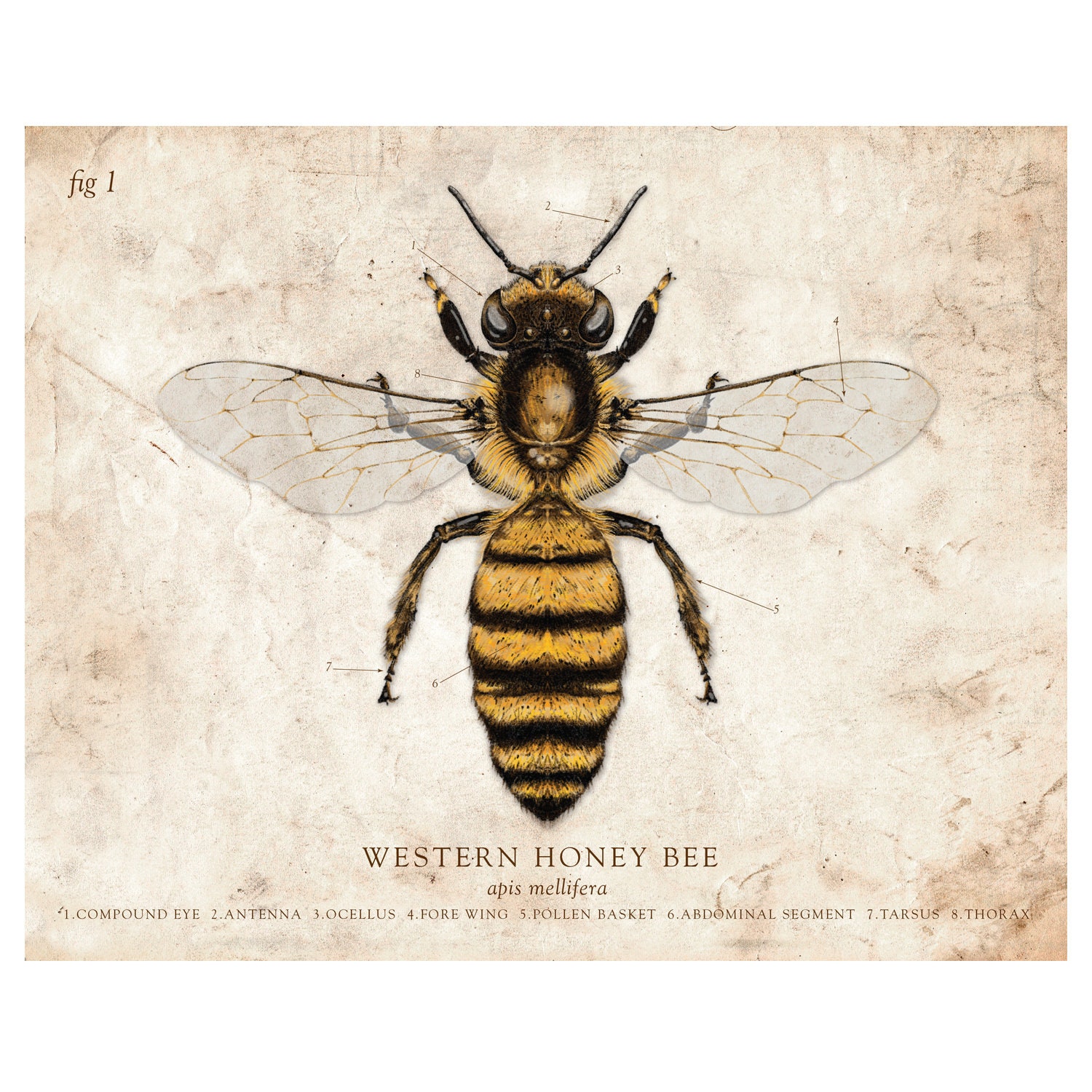This detailed image is a full-color rendering of a Western honeybee, Apis mellifera, and is set against a cream, stone-textured backdrop that appears slightly wrinkled. Positioned centrally in a landscape layout, the bee is illustrated from an overhead perspective, showcasing distinctive yellow and black markings, open wings, and its antennae, eyes, six legs, and thorax. Lines and arrows extend from the bee to indicate eight numbered anatomical features: one for the compound eye, two for the antennae, three for the ocellus, four for the forewing, five for the pollen basket, six for the abdominal segments, seven for the tarsus, and eight for the thorax. These numbers correspond to labels at the bottom of the image. At the top left corner, in brown text, it reads "Fig 1," echoing the scientific and intricate nature of this illustration.